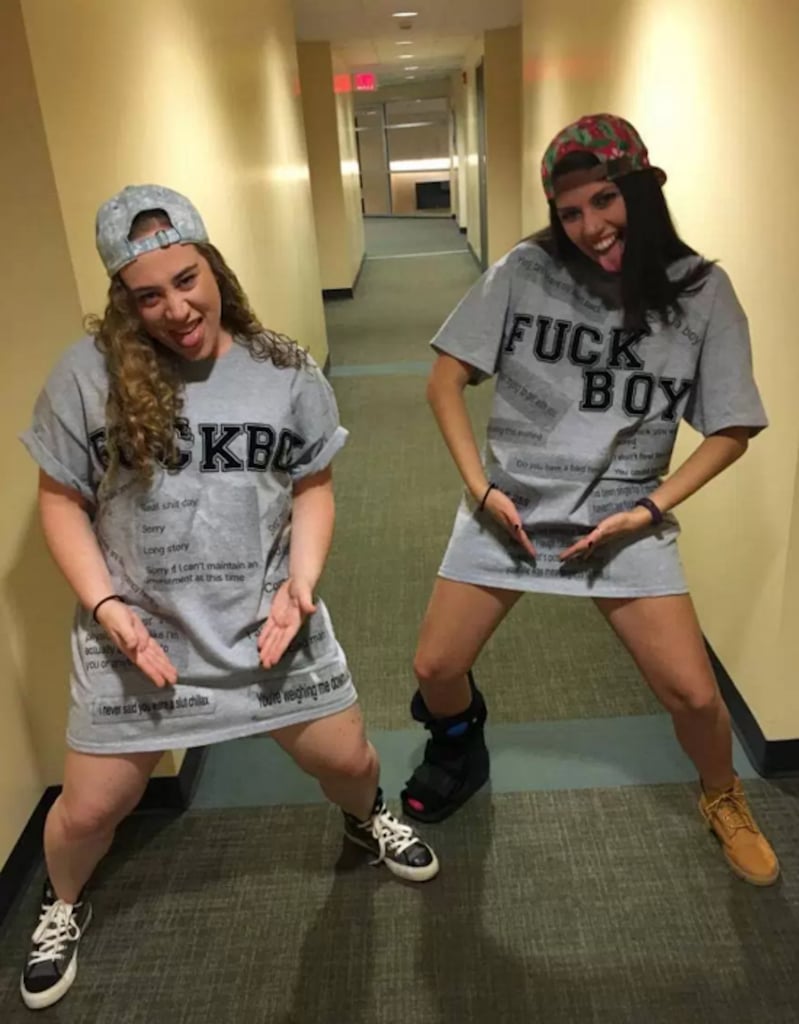In a dimly-lit hotel hallway with eggshell yellow walls and old brown carpet, two young women stand side by side, each wearing a backward baseball cap. The girl on the left dons a gray cap and black and white Converse sneakers, with her curly blonde hair peeking out. The girl on the right sports a multicolored cap, a brown loafer on her left foot, and a black medical boot cast on her right foot, indicative of an injury. Both girls are clad in oversized gray t-shirts that extend down to their thighs, leaving their legs bare, and display an obscene term in bold black font that reads "F-U-C-K boy." They are pulling playful expressions with their tongues sticking out and making a V-shape with their hands pointing downwards, each girl's hands are separated but symmetrically posed. An exit sign is visible at the end of the hallway, casting a soft glow on their cheeky appearances.